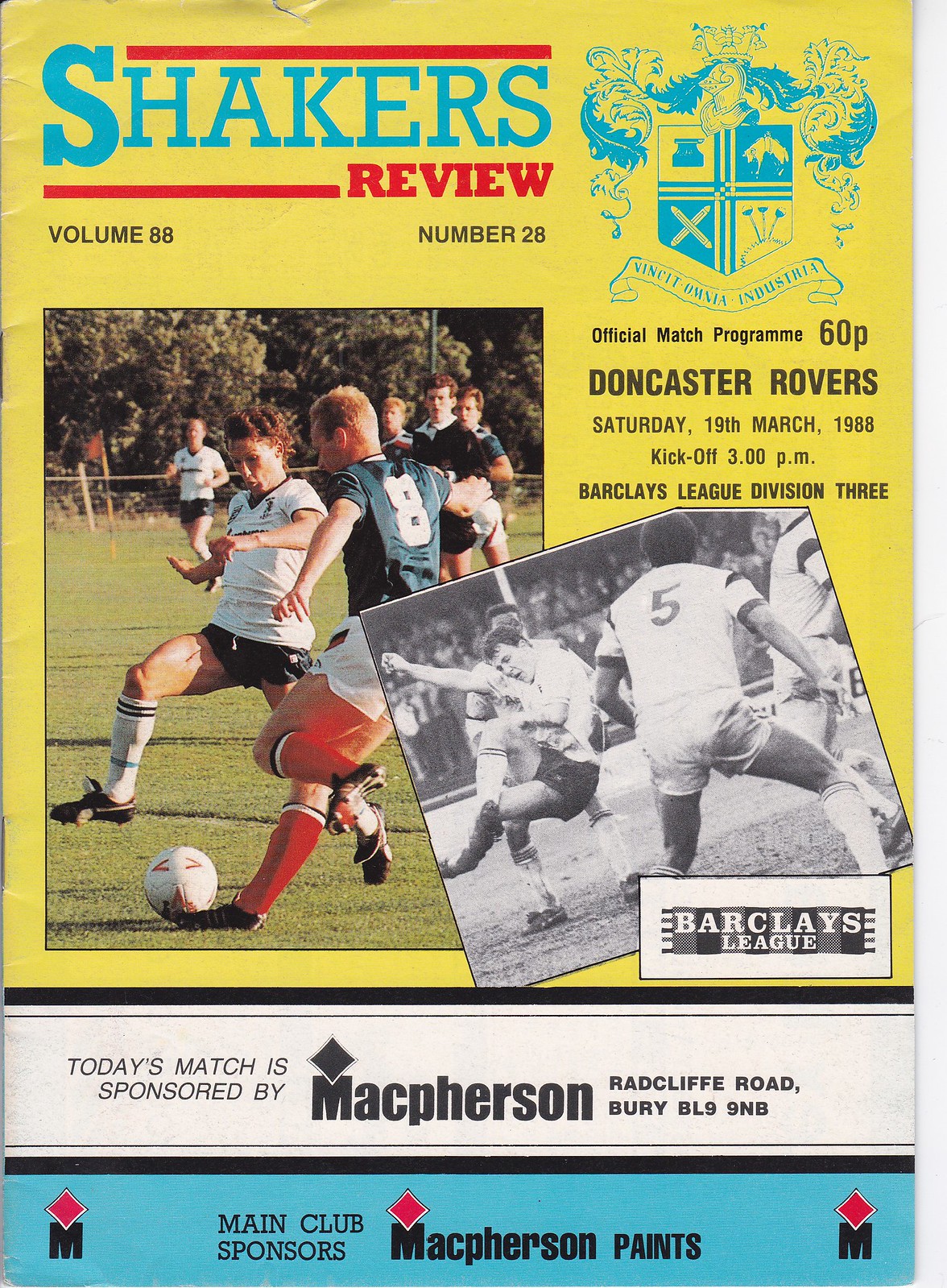The cover image of the Shaker's Review, volume 88, number 28, serves as the official match program for the Doncaster Rovers' football game against Bury on Saturday, March 19th, 1988. Priced at 60 pence, this vintage program announces a kickoff at 3 p.m. for the Barclays League Division III match. Dominating the upper right is an elaborate blue crest featuring a medieval knight's helmet, feathers, and the Latin phrase "Vincent Omnia Industria." The program's top section is yellow, presenting the text and logo prominently.

Two photographs capture the action: on the left, a full-color image portrays a player in a white shirt and black shorts attempting to kick the ball, challenged by an opponent in a black shirt and white shorts on a green field. On the right, a black-and-white photo held at an angle shows several players contesting for the ball, with one player, numbered 5, having his back to the viewer. Below these images, a white stripe and a blue stripe at the bottom of the cover contain the text "Barclays League" and "Today's match is sponsored by McPherson, Radcliffe Road, Bury, BL9 9NB," with the main club sponsor noted as McPherson Paints.